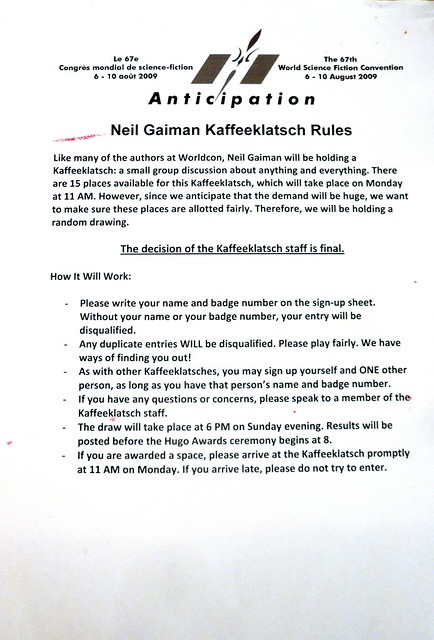In the image, there is a printed document titled "Neil Gaiman Kaffee Klatsch Rules" related to the 67th World Science Fiction Convention (Worldcon) held from August 6-10, 2009, also referred to as Anticipation. The document, primarily in English but with some details in French (L.E. 67E, Congress Mondial to Science Fiction 6-10 A.O.U.T. 2009), outlines a small group discussion session led by author Neil Gaiman, referred to as a "Kaffee Klatsch." There are 15 available spots for this session, scheduled for Monday at 11 a.m.

Noting the high demand, the organizers have decided to allot spots through a random drawing. Participants must write their name and badge number on the sign-up sheet; entries lacking this information or containing duplicates will be disqualified. The rules emphasize playing fairly, with a warning that the organizers have the means to detect cheating. Attendees can sign up themselves and one other person, provided they have the person’s name and badge number. The drawing will be held at 6 p.m. on Sunday evening, with results posted before the Hugo Award Ceremony at 8 p.m. If selected, participants must arrive promptly at 11 a.m. on Monday; latecomers will not be admitted. The document encourages any inquiries to be directed to the Kaffee Klatsch staff. The top left and right corners of the document highlight the event's title and date details in both English and French.